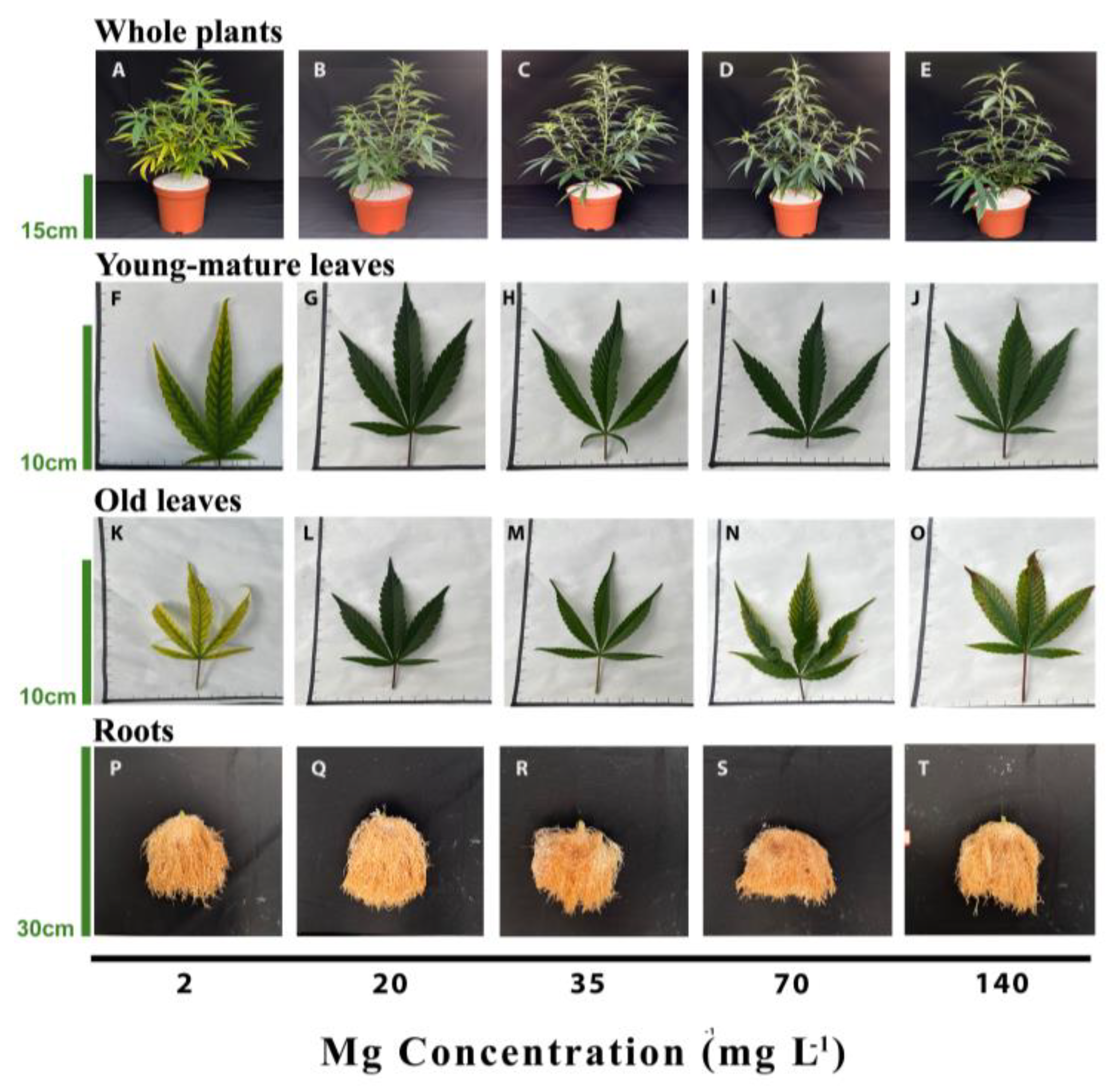The image showcases a detailed layout of plant development stages against a plain white background. It is organized into four rows and five columns, totaling 20 thumbnails. The top row, labeled "Whole plants" in black print, features five images (A to E) of a plant in a red pot, showing progressive growth stages. To the left of these images, in green print, it indicates 15CM. The second row is titled "Young mature leaves" and includes close-up shots of young leaves labeled F to J, marked 10CM to the left. The third row, "Old leaves," displays older, smaller leaves labeled K to O, with a 10CM label to the left. At the bottom, the row titled "Roots" contains images of roots, labeled P to T and indicated as 30CM to the left. Along the very bottom of the image, there’s a black bar listing the numbers 2, 20, 35, 70, and 140. Below this bar, it states "Mg concentration (MgL^-1)" in black print, detailing the concentrations used in the study.